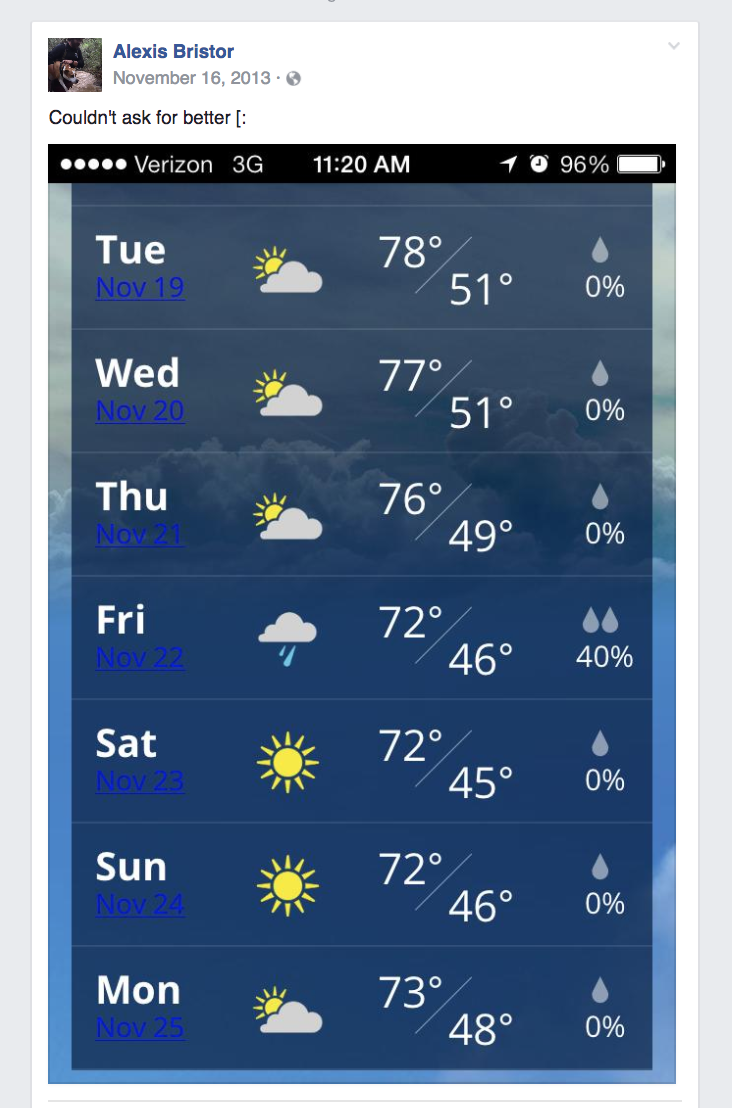**Detailed Caption**:
This image is a screenshot of a public Facebook post made by Alexis Bristor on November 16, 2013. In the post, Alexis's profile picture is visible as an avatar. The post reads, "Couldn't ask for better :)" using keyboard characters to form a smiley face instead of an emoji. The main content of the screenshot is a weather forecast covering the period from Tuesday, November 19 to Monday, November 25.

The forecast indicates mostly sunny weather throughout the week, with the exception of Friday, November 22, which shows a 40% chance of rain. The temperature for the week ranges from the lower to upper 70s Fahrenheit, with the highest temperature being 78°F on Tuesday, November 19. For both Saturday, November 23 and Sunday, November 24, sunny weather is expected. 

Additional elements in the screenshot include a battery icon showing 96% at the top right corner and the time displayed at the center of the status bar as 11:20 a.m. The status bar itself has a black background. This weather forecast screenshot is included as part of Alexis's Facebook post.